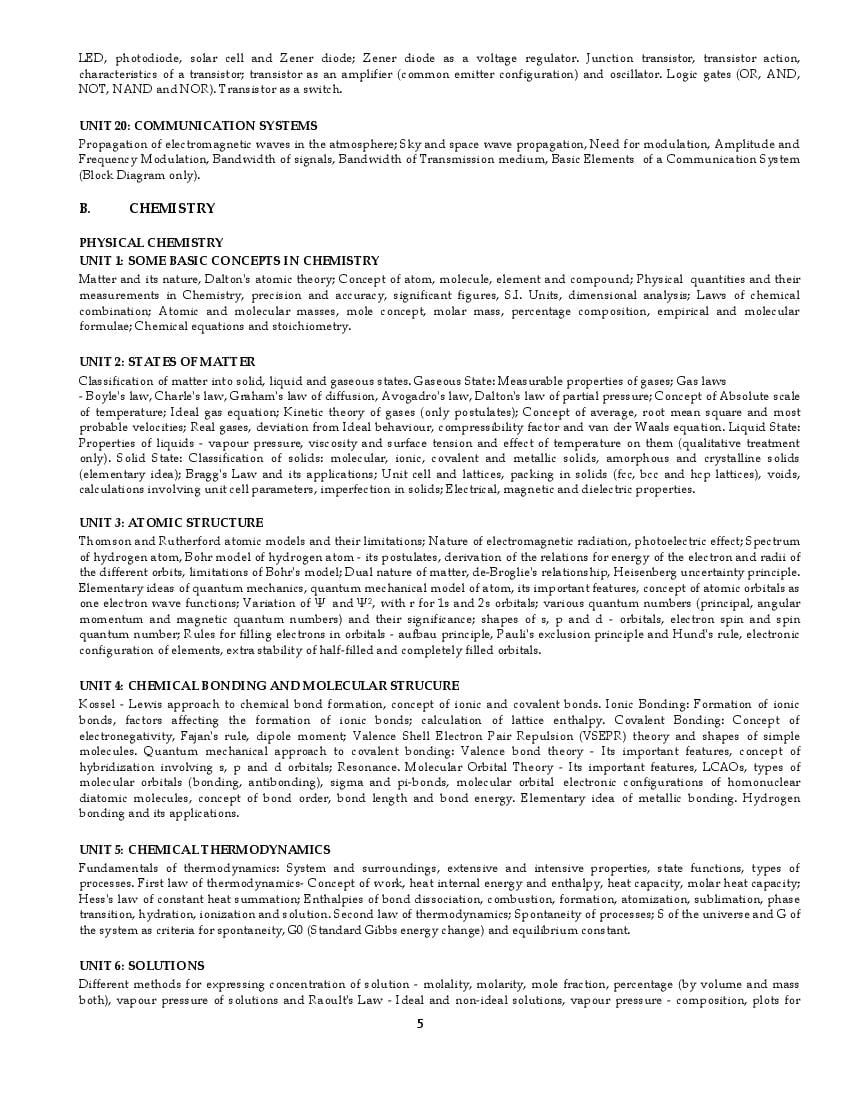The image displays a comprehensive schematic covering various electronics and communication systems concepts, along with fundamental chemistry principles. 

In the electronics section, it illustrates a range of components including text LEDs, photodiodes, solar cells, and Zener diodes (notably used as voltage regulators). A junction transistor is highlighted with specific mentions of transistor action, current transistor amplifiers, common configurations, and oscillator logic gates such as OR, AND, and NOT gates. Additionally, there is a depiction of transistors functioning as switches and their application in Unit 20 communication systems, emphasizing the propagation of electromagnetic waves in the atmosphere. 

The science section delves into concepts of propagation, neural modulation, amplitude, and frequency modulation, and the bandwidth of signals. There's an in-depth look at the governmental role in communication technologies and how they integrate with the technological advancements in chemistry.

Moving to the chemistry portion, the image introduces Unit 1 basics, detailing processes in chemistry, the nature of matter, molecular concepts, elements, and compounds. It further explains physical quantities and their measurements, with emphasis on positional accuracy, significant figures, SI units, and dimensional analysis. There’s a mention of the laws of chemical combination, albeit briefly.

Overall, the image provides a detailed interplay of electronics and communication system technologies alongside foundational chemistry principles, illustrating the complex interrelation in these scientific fields.